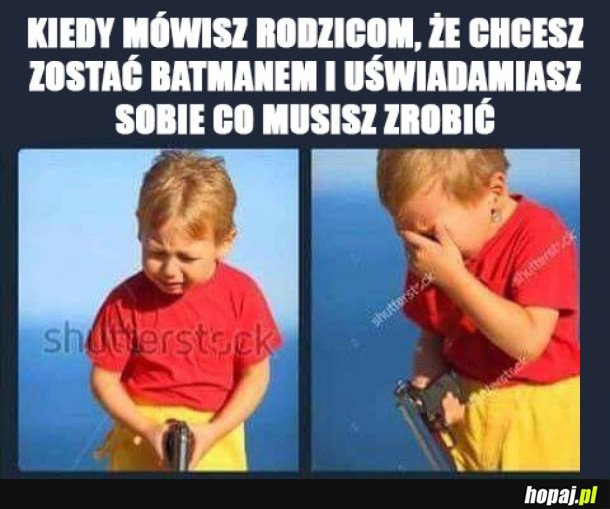This image features two photos of the same young, blonde-haired toddler against a solid black background. The top of the image contains three lines of white, uppercase text in a foreign language, possibly German or Polish. The two main photos occupy the middle and bottom sections of the image. In the left photo, the toddler, dressed in a short-sleeved red shirt and yellow shorts, faces the viewers but looks down, appearing distressed and crying. He holds a dark gray object, resembling a gun, in both hands. The word "Shutterstock" is watermarked across this photo. In the right photo, the toddler is shown from a side angle, with his left hand covering his face as he continues to cry. He holds the same object in his right hand. The background behind the boy transitions from dark blue to light blue, adding to the overall somber mood conveyed by his distress.